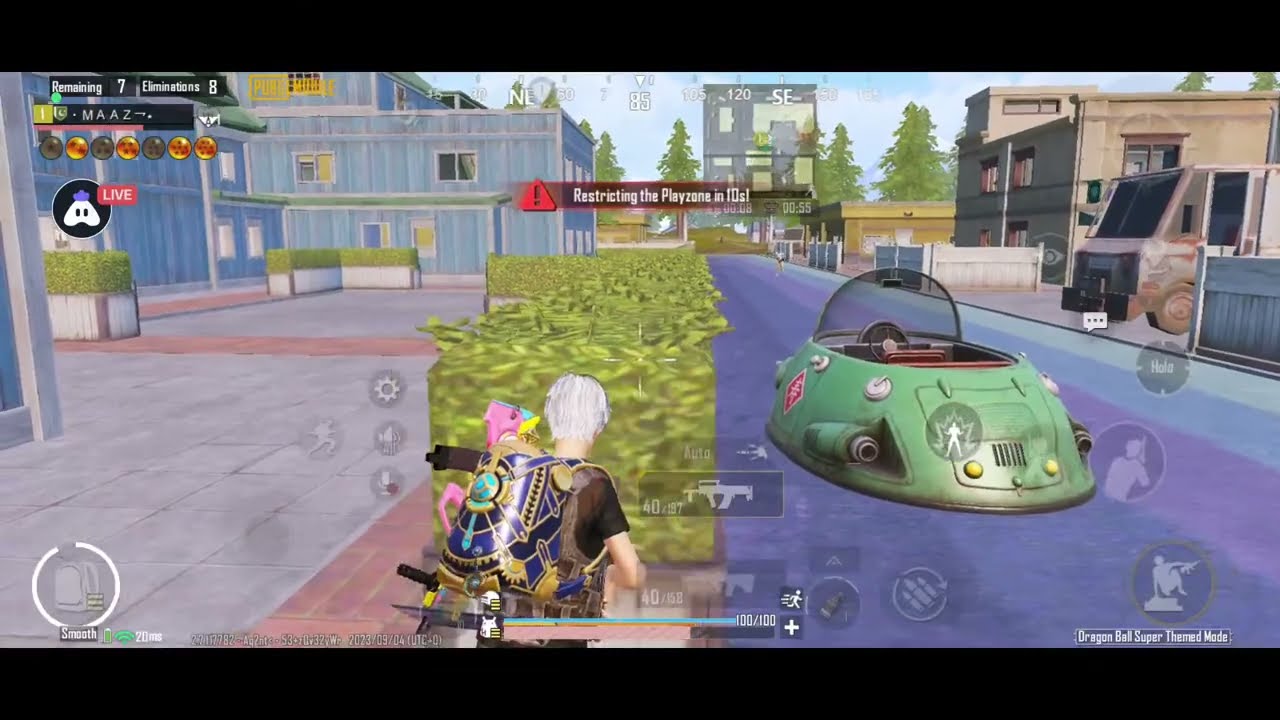This is a highly detailed screenshot from a video game, featuring a richly textured 3D environment. In the foreground, a character stands at the bottom center of the screen. He has distinctive silver or white hair and wears a vest along with a backpack adorned with various colorful gears and accessories, including hues of purple, green, blue, and black. In front of him, there is a block of grass, and to the right, a river containing a green hovercraft-like vehicle equipped with a steering wheel, two engines, and an exhaust or trunk area.

The scene also includes a road on the right bordered by buildings. Among these structures is a factory-like building on the left, and beside the road is a gray truck resembling a mail truck. Hedges and what looks like a brick sidewalk add to the urban landscape. The mid-ground depicts more buildings, with some appearing futuristic.

Overlaying the game scene are various UI elements, including a transparent gun image, ammunition indicators, and a selection interface for different guns. A life bar is visible at the bottom of the screen, while on the upper left, buttons and a score display read '7 to 8'. A red triangle with an exclamation mark in the middle alerts players with the message, "restricting the play…". Additional symbols and texts, like a 'live' indicator with a controller icon, appear on the extreme left, combined with other unreadable graphical elements and some trees in the background.